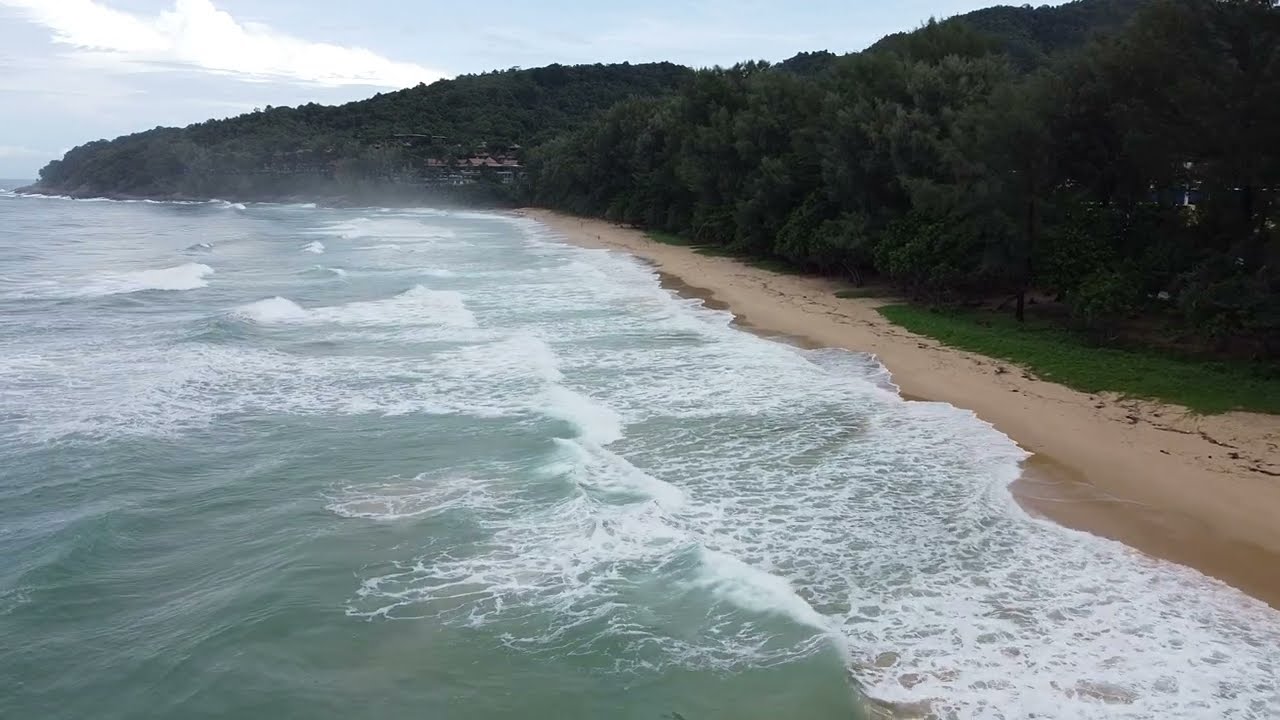This is a detailed aerial photograph of a coastline taken from a high vantage point, likely a drone. The image captures a natural seashore scene. On the left side, the sea showcases a dark aqua or turquoise hue, with frothy white waves breaking onto the shoreline. The water becomes almost white and highly oxygenated as it nears the sandy beach. The beach features a curved line, wider on the right side and narrowing toward the back center of the photograph, covered in rich brown sand. Beyond the beach, the hills are densely forested with dark green trees, creating a striking contrast with the lighter, pastel blue sky above. A narrow strip of white and puffy clouds can be seen hanging in the top left corner of the image. Additionally, there are some buildings nestled within the dense woods, visible in one portion of the hillside, while the rest of the area remains predominantly natural and untouched. Overall, this scene, captured in a landscape orientation, epitomizes photographic realism and representationalism.